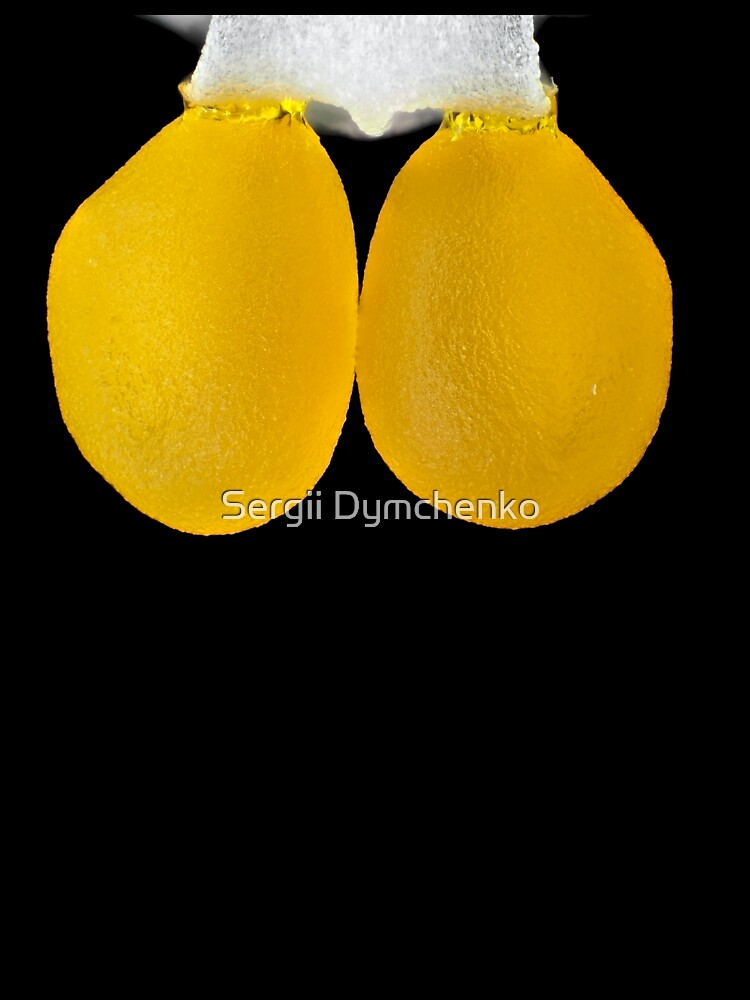This image features a stark, jet-black background with a mysterious object suspended from the top center. The object comprises a textured, white foamy material that forms a rectangular shape, appearing almost see-through and flipped up at the center. From this white section hang two bright, yellow bulbous sacs, resembling lemons, both sporting golden ribbons around their tops. These yellow bulbs are nearly transparent against the dark backdrop. The name "Sergei Dimchenko" is prominently displayed in white lettering just beneath these sacs, acting like a watermark. Despite the primarily black and blank lower half of the picture, a small, blurred white shape is faintly visible to the left of the main white structure, suggesting there may be more hidden details.